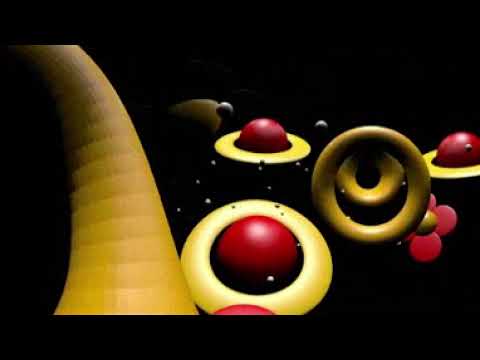The image is a 3D-rendered, surreal scene with a space-like vibe and abstract designs. Dominating the left side, a yellow corded tube extends from the bottom and curves up to the upper left corner, featuring horizontal lines running across its surface. On the right, three red spheres, reminiscent of planets with yellow rings similar to Saturn's, float against a pitch-black background. Among these are two golden yellow rings, one larger and one smaller inside it. Nestled between these planetary objects is a small pink flower with four petals and a yellow center. Tiny white dots trail from the planets, adding to the ethereal atmosphere. It appears to be a piece of digital or computer-generated art, evoking a sense of floating in the cosmos.